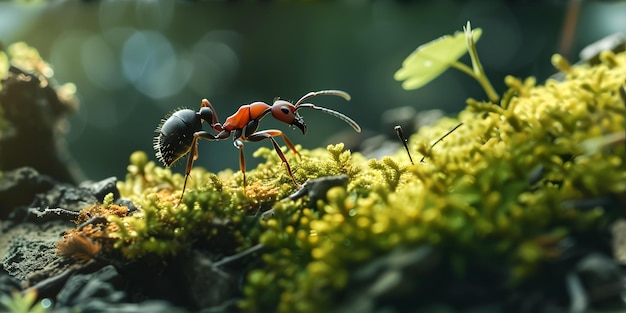This highly detailed, photorealistic image features a close-up of a reddish-orange ant with pomegranate-colored body and black accents, standing and walking through lush green moss. The ant’s six legs, two downward-facing antennae, and the black, slightly hairy, bulbous end of its abdomen are distinctly visible. It is situated within a vibrant landscape of green vegetation, possibly growing on the root or branch of a tree, with a small leaf and some plant material nearby. The forest floor underneath reveals bits of rock and dirt. The background is artistically blurred using a bokeh effect, emphasizing the ant as the focal point. Sunlight flares from the top left corner add a natural touch to the vividly green and fresh appearance of the scene.